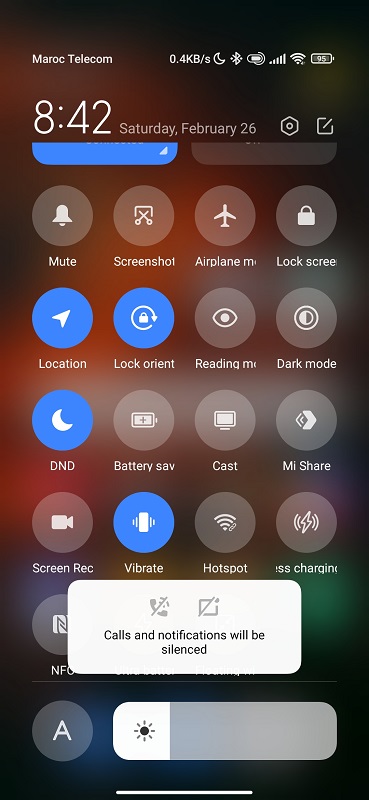The image showcases a smartphone screen with various icons and information. In the upper left-hand corner, the screen displays the text "Maroc Telecom" in white font, indicating the telecom provider. Adjacent to this, several status icons appear, including a data speed of 0.4 gigabytes per second, a moon symbol, Wi-Fi signal strength, cell signal bars, and battery life, all rendered in white.

Below these status indicators, on the left-hand side, the screen shows the time as 8:42 and to the right, the date is displayed as Saturday, February 26th. Additionally, two small icons sit to the right of the date and time; one resembles a hexagon and the other looks like an edit symbol.

Further down, a grid of 16 circular buttons appears, organized in a 4x4 layout. Each button represents a specific function and features an icon related to its action. The buttons are categorized as follows:

- **First row:** Mute, Screenshot, Airplane Mode, Lock Screen
- **Second row:** Location, Lock, Screen Orientation, Reading Mode
- **Third row:** Do Not Disturb (DND), Battery Saver, Cast, My Share
- **Fourth row:** Screen Recording, Vibrate, Hotspot, Wireless Charging

Most of these buttons are gray with a white icon inside, except for the Location, Lock, Screen Orientation, DND, and Vibrate buttons, which are blue with a white icon, indicating these options are currently activated.

Beneath the fourth row of buttons, there is a rectangular white pop-up box with black text that reads, "Calls and notifications will be silenced." Below this notification, the screen displays a brightness adjustment slider, set at approximately 20 to 25 percent brightness.